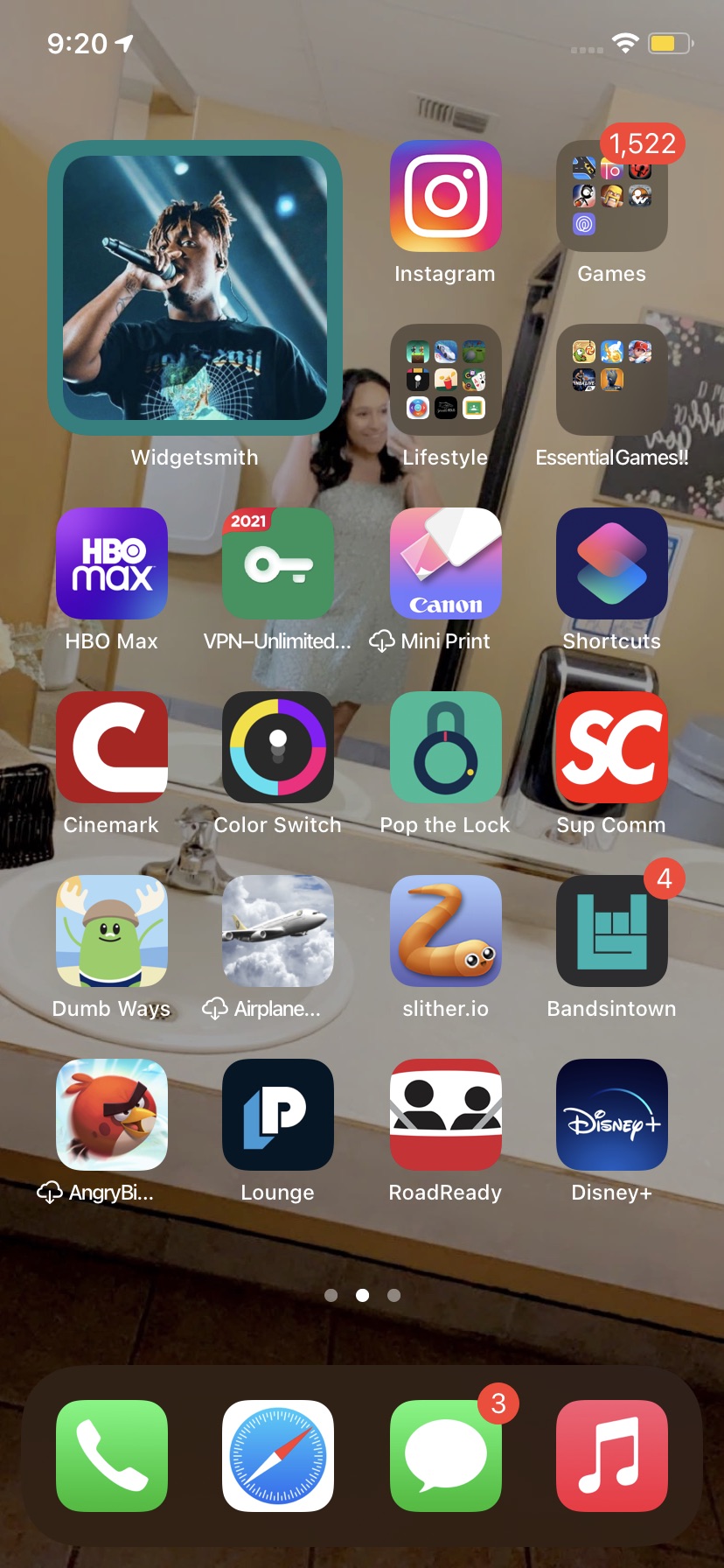This screenshot captures the home screen of an iPhone. The wallpaper appears to be a real photograph taken by the user, featuring a reflection of a woman, possibly Asian or Latina, with dark hair. She is wearing a white dress that seems to have a lace-like pattern, possibly due to shadowing. The woman is smiling while taking a selfie in a bathroom, the setup of which is discernible from the white bathroom counter with a porcelain sink on the left, accompanied by a metallic silver faucet.

At the top left of the screen, the time is displayed in white text as 9:20. An arrow icon next to the time indicates that location services are active. The top right shows a series of four grayed-out dots, indicating that there is no cell service, alongside a Wi-Fi icon with three arcs suggesting a strong signal, and a battery icon that is about two-thirds full and displayed in yellow.

There is a larger icon at the top left with a teal background featuring a photograph of a black man holding a microphone, singing at a concert while wearing a black T-shirt with a graphic design. The text below this photo reads "Widget Smith."

The home screen further consists of four additional icons situated to the right of the Widget Smith widget, 16 app icons arranged in a grid below the widget, and an additional row of four icons at the very bottom.